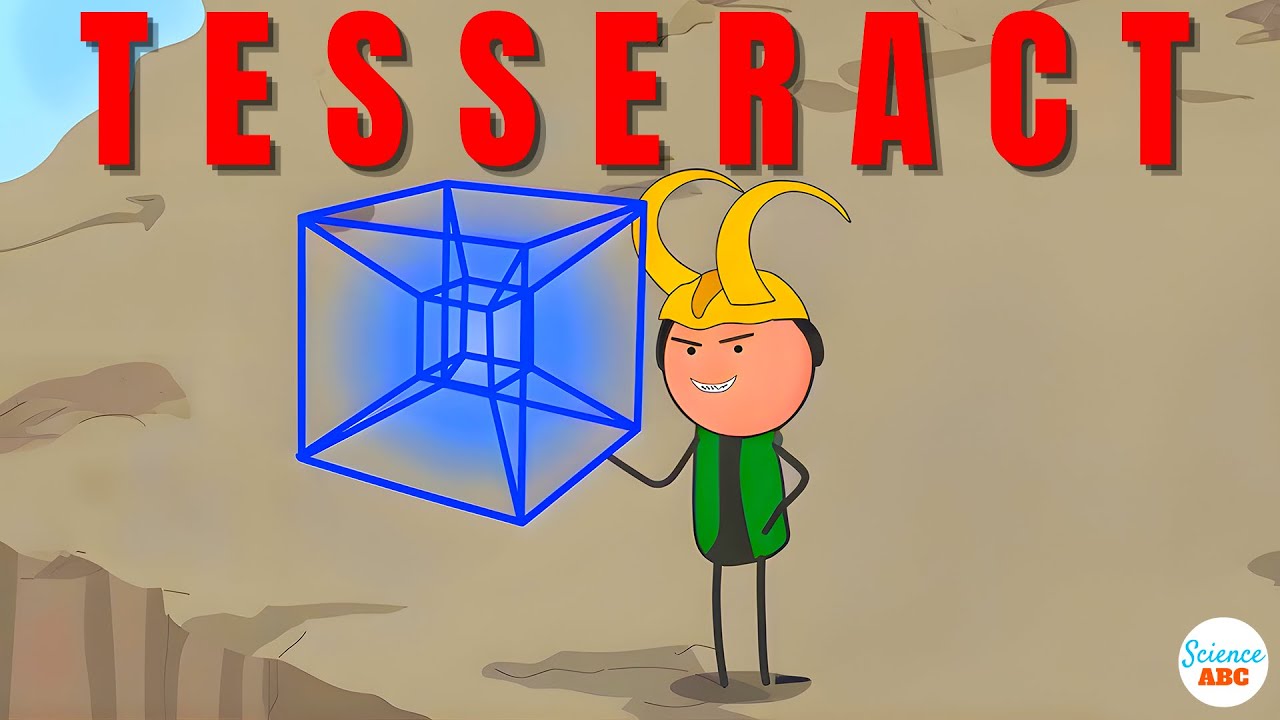This colorful and dynamic cartoon image prominently features a child-like version of Loki, depicted as a stick figure character with a big, round beige-peach head, black eyes, straight black eyebrows, and a crescent-shaped smile with braces. He is donned in Loki's iconic attire - a green shirt with black accents, a flowing green cape, and a distinctive golden helmet adorned with two large, backward-arching horns. In one of his small black hands, he holds a glowing, translucent blue tesseract, which is intricately outlined with connecting lines to form a smaller cube within the larger cube.

The character stands proudly on a brown, rocky plateau, near the edge which suggests a drop-off on the left side of the image. Above him, in the upper part of the scene, the word "TESSERACT" spans across in big, bold red letters. At the bottom right corner, a white circle encloses the words "Science" written in blue and "ABC" in orange, possibly indicating either the network or the name of the show. The background and setting, combined with the elaborate details of Loki's youthful and cheerful representation, brings out a whimsical and adventurous essence to this imaginative and detailed animation.